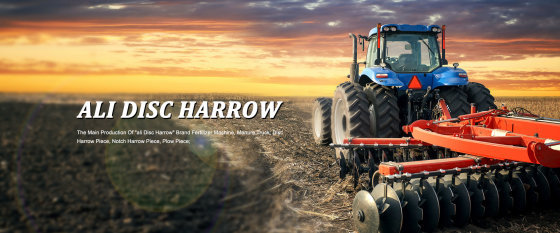The advertisement photo features a blue, heavy-duty farm tractor in the lower right corner, equipped with an orange slow-moving vehicle triangle in the center. The tractor, which has two large black tires on each side, is pulling a disc plow and is actively plowing a broad, open field. On the left side of the image, center-aligned, the words "Alley Disc Harrow" are prominently displayed in white letters, with smaller subtext beneath it indicating "the main production CF-48 Disc Harrow." The horizon above the field showcases a striking sunset with hues of orange, yellow, and violet, contributing to the traditional, picturesque late afternoon setting.